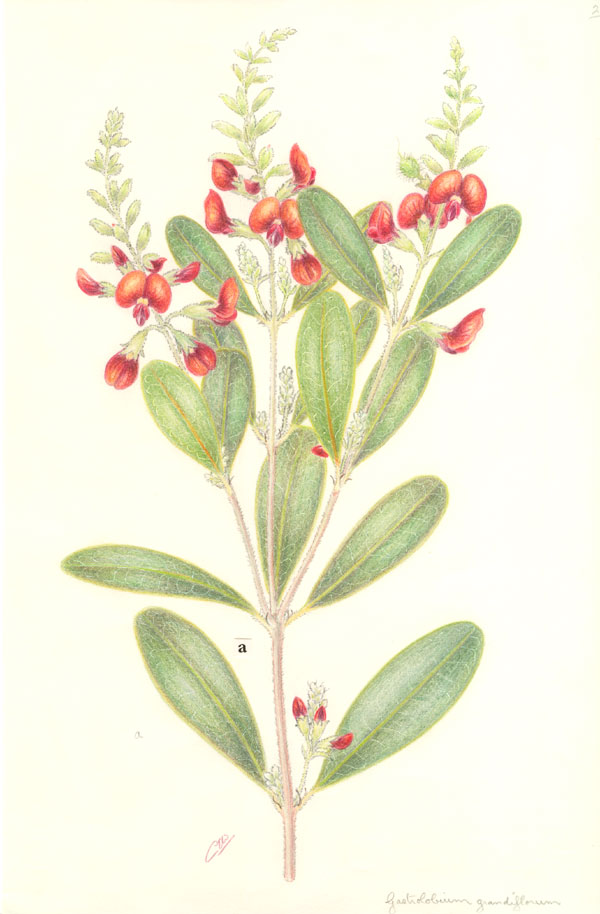The image is a detailed rendering or illustration of an elegant, tall, vertical flowering plant, set against a pure white background for dramatic effect. The plant features approximately 12 to 14 long, slender, green leaves, each characterized by a single central vein. At various points along the stem, there are multiple small, decorative, red buds. Some of these red buds resemble puffy petals but do not open into full flowers. The top part of the plant also has additional green leaves among the red buds, creating a lush and vibrant appearance. At the bottom of the image, there is small text that is difficult to read, likely indicating either the plant's Latin name or the artist's signature. This artistic depiction showcases the plant in a style reminiscent of botanical illustrations found in magazines or educational books.